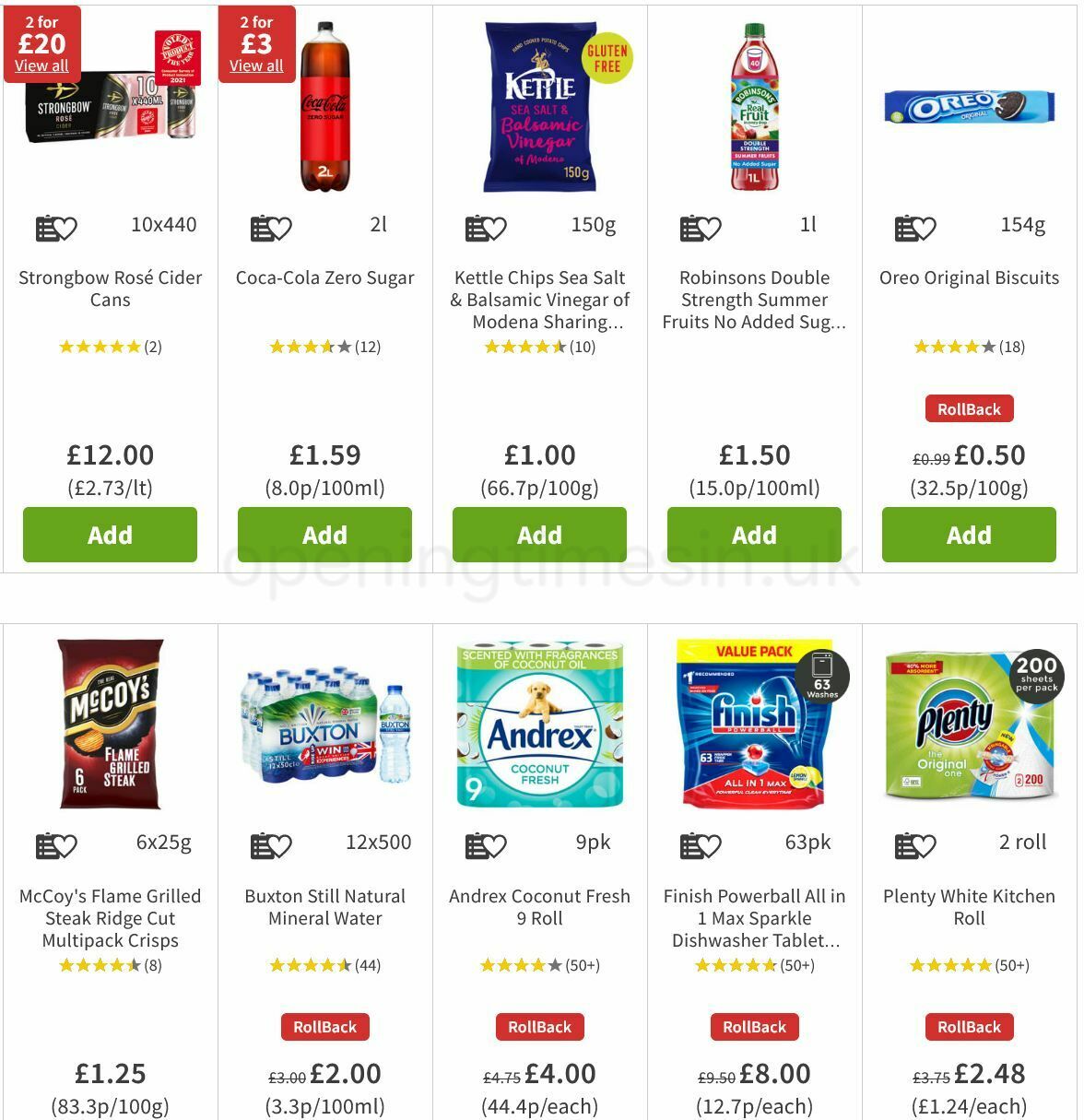In this image, we can see a variety of grocery store items neatly arranged in a grid formation. There are a total of 10 items displayed, divided into two rows of five. The top row displays items clearly, each with a green "Add" button labeled below them, containing white text. The bottom row is partially cut off due to the limited view of the screenshot, making its "Add" buttons invisible.

Starting from the top left and moving right, the following items are shown:

1. **Strongbow Rosé Cider Cans**:
   - Rating: 5 stars, based on 2 reviews.
   - Price: £12.
   - Green "Add" button below the cider cans.
  
2. **Coca-Cola Zero Sugar**:
   - Rating: Approximately 3.5 stars, based on 12 reviews.
   - Price: £1.59.
   - Green "Add" button below.

3. **Kettle Chips Sea Salt and Balsamic Vinegar of Modena**:
   - Rating: 4.5 stars, based on 10 reviews.
   - Price: £1.
   - Green "Add" button below.

4. **Robinsons Double Strength Summer Fruits, No Added Sugar**:
   - Rating: Not explicitly mentioned, but implied good quality.
   - Price: £1.50.
   - Green "Add" button below.

5. **Oreo Original Biscuits**:
   - Rating: 4 stars, based on 18 reviews.
   - Price: £0.50.
   - Green "Add" button below.

In the bottom row, from left to right:

6. **McCoy's Flame Grilled Steak Rich Cut Multi Crisps**:
   - Rating: 4 stars, based on 8 reviews.
   - Price: £1.25.

7. **Buxton Still Natural Mineral Water**:
   - Rating: 4.5 stars, based on 44 reviews.
   - Price: £2.
   
8. **Andrex Coconut Fresh 9 Roll**:
   - Rating: 4 stars, based on 50+ reviews.
   - Price: £4.
   
9. **Finish Powerball All-in-One Max Sparkle Dishwasher Tablets**:
   - Rating: 5 stars, based on 50+ reviews.
   - Price: £8.
   
10. **Plenty White Kitchen Roll**:
    - Rating: 5 stars, based on 50+ reviews.
    - Price: £2.48.
   
The image displays the top selection of the grocery items, highlighting various products along with their ratings, review counts, and pricing.